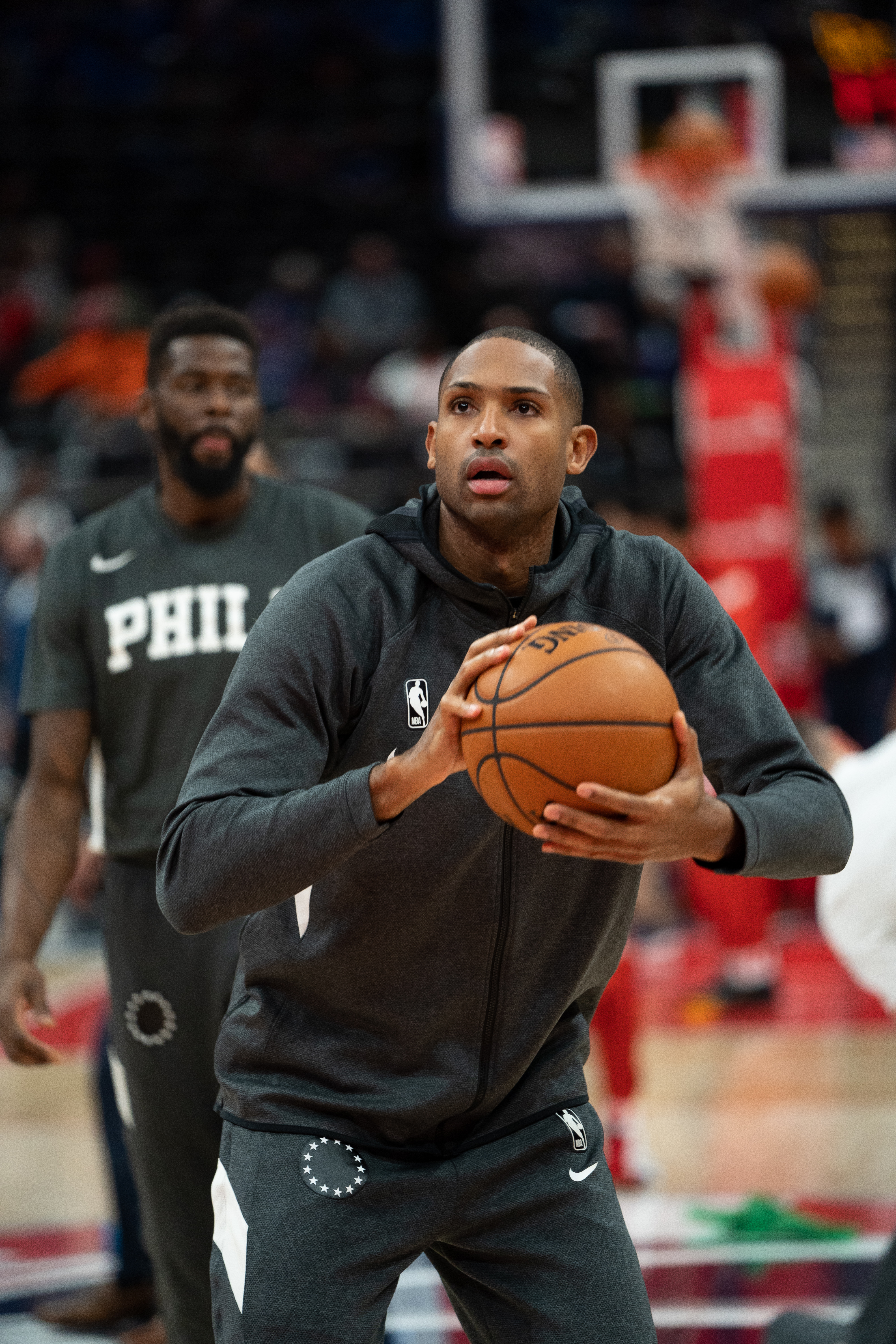In the image, a basketball player, dressed in a gray hoodie with the NBA logo, Nike logo, and a circle of stars logo, practices holding a basketball with both hands. He's looking upwards towards the top left, seemingly aiming at the basketball hoop. The player also wears matching gray pants with similar logos. Behind him stands another player in a short-sleeved gray shirt with the Nike logo and the letters "P-H-I-L" on the front, also wearing the same gray pants. Both men appear to be professional players, possibly warming up before a game. The scene features a basketball court with a hoop in the background and spectators seated in the stands, watching the practice. The focus is on the well-coordinated practice session, highlighting both players' preparation and teamwork.